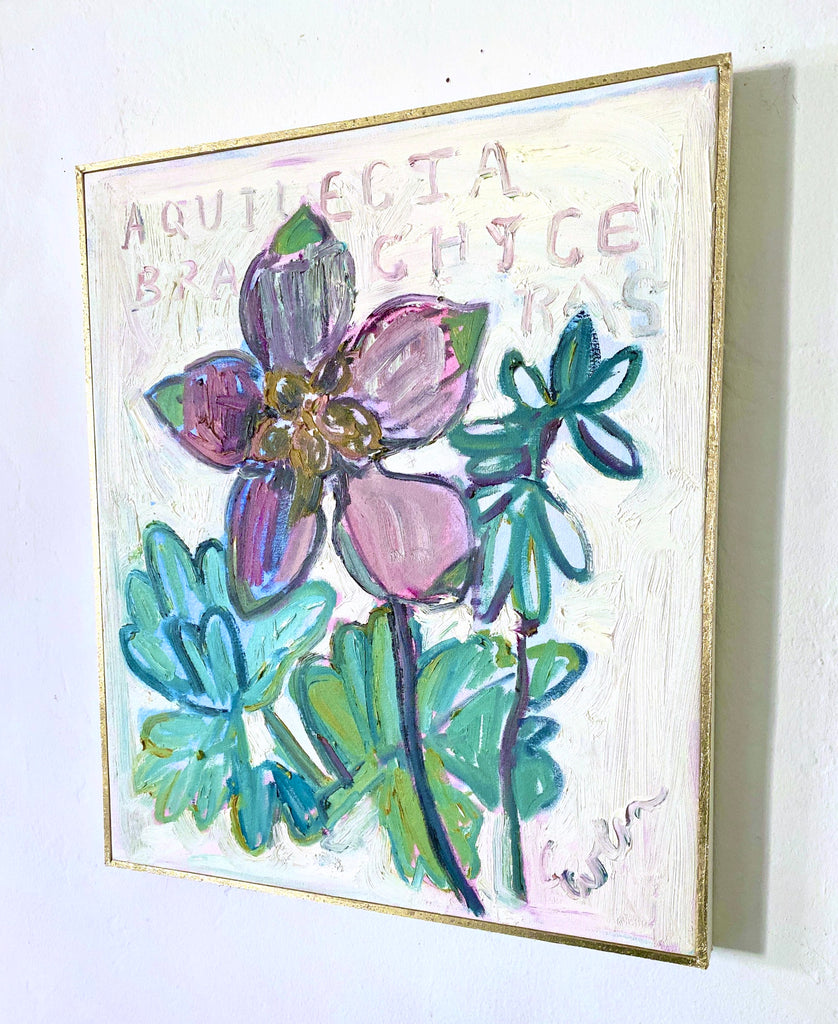The painting depicted in the vertical rectangular image is a square canvas framed with a thin, shiny gold trim, hanging against a textured white wall. The light source from the left casts a noticeable shadow on the right side of the frame. The canvas showcases an expressive, painterly style with prominent brush strokes. The artwork predominantly features a central purple flower with green-tipped petals, set against a mostly white background. Surrounding the flower are additional floral elements in colors including various shades of green and hints of blue and pink. The overall composition has a childlike quality. At the top of the painting, faint text in a light purple color reads what appears to be "Aquilecta" or "Aquilechia," followed by "BRACTCE RAS," potentially a scientific name for the flower. The painting bears a signature in black in the bottom right corner, which appears somewhat scribbled.